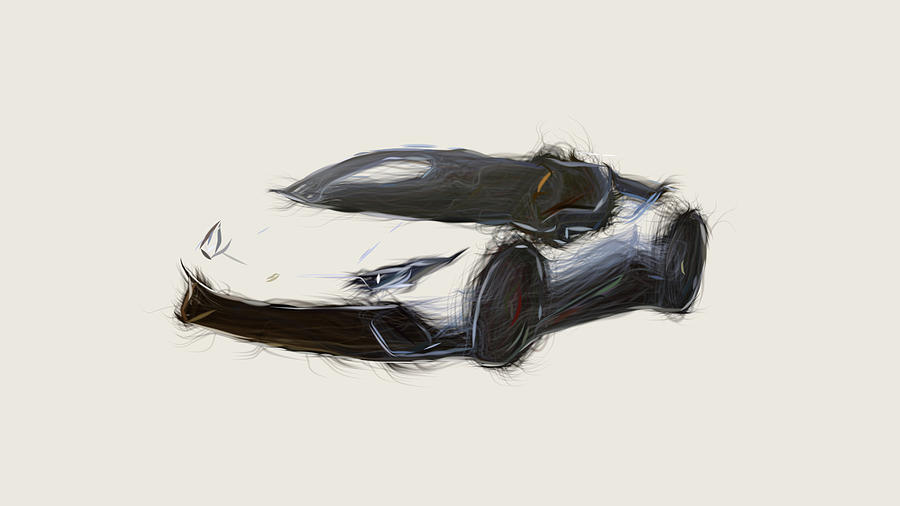This image is a detailed and dynamic charcoal sketch of a sleek white sports car, likely meant to resemble either a Lamborghini or a Ferrari. The car is portrayed with a low stance, emphasizing its aerodynamic and aggressive design, including black accents such as the wheels, grille, and roof. The windows are tinted, and there's a distinct glare on one, adding to its aggressive appearance. The sketch is on an ivory or white background, devoid of any added scenery, focusing solely on the vehicle. The drawing appears messy or distorted, created with charcoal, pencil, or possibly a brush, giving it a windswept, in-motion feeling with lots of wisps and smudges. Notably, there are tiny specks of red and hints of the Ferrari logo with its yellow design. The sketch's roughness and smudged lines contribute to the impression of speed and motion, as though the car is racing off the page.